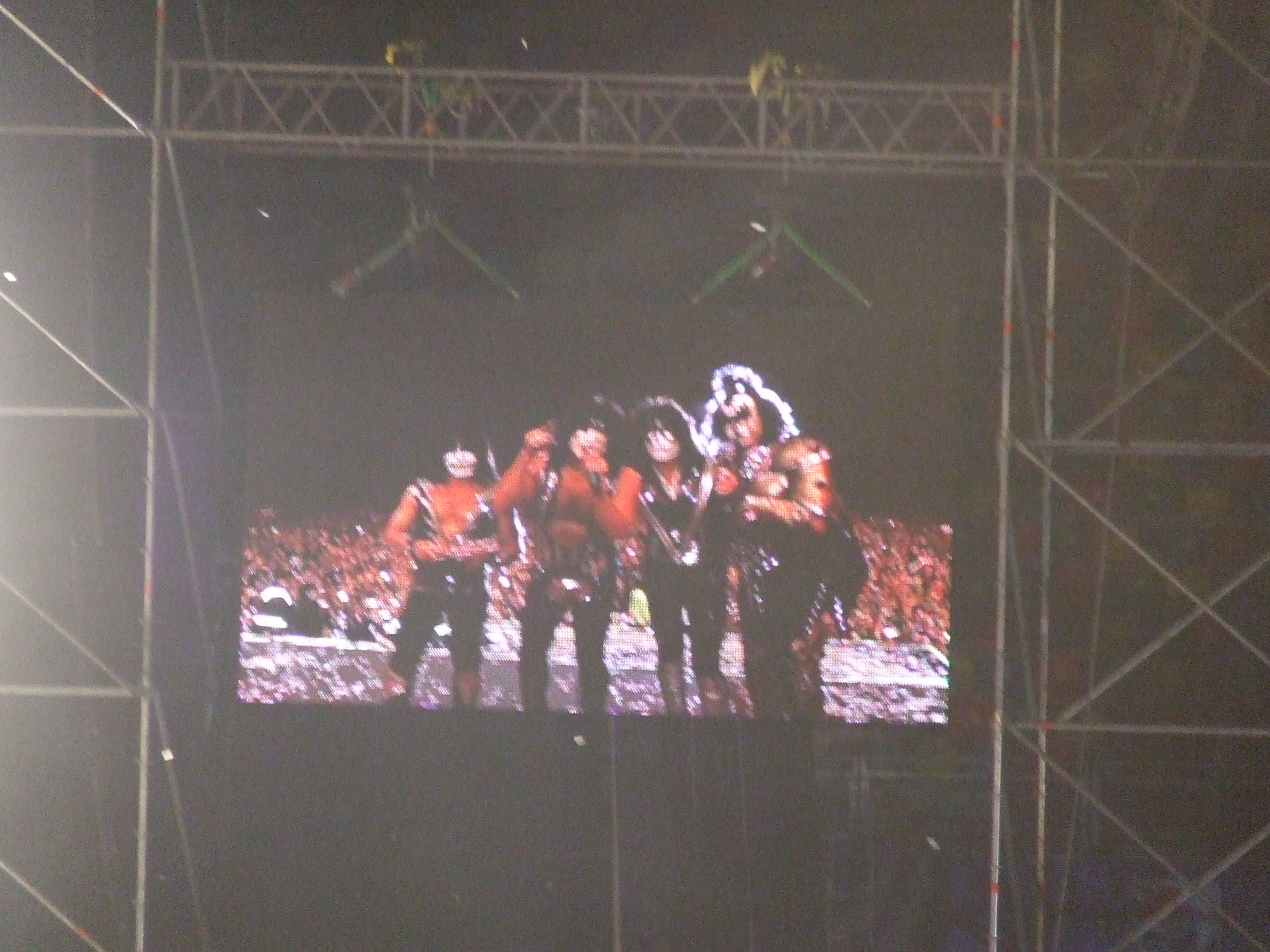The photograph, taken in low light with a somewhat hazy and blurry quality, captures a nighttime outdoor concert. The image features a black background and centers on a large jumbotron screen displaying the band KISS. The screen is part of a stage setup supported by extensive metal scaffolding, including metal frames on the sides and a catwalk above. The band members, standing in a row and facing the camera, are dressed in characteristic leather outfits with their faces painted in the iconic white face paint. Behind them, a large crowd is faintly visible. The entire scene is surrounded by a dark, moody atmosphere, enhancing the concert's intense and gothic ambiance.